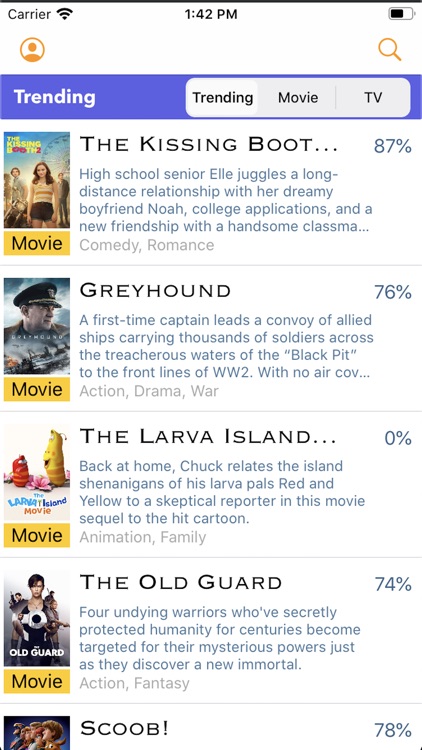Here is a detailed and polished caption for the image described:

---

A screenshot of a cell phone display at 1:42 PM showcases a half-filled battery icon and a generic placeholder for the carrier name. At the top of the screen, a blue bar labeled 'Trending' in white text highlights the current popular content. Below, a section titled 'Trending Movies and TV' presents a list of featured films with accompanying images.

1. **The Kissing Booth**: A high school senior named Ellie juggles a long-distance relationship with her dreamy boyfriend Noah, college applications, and a blossoming friendship with a classmate. This comedy-romance film boasts an 87% rating.
   
2. **Greyhound**: A first-time captain undertakes a hazardous journey, leading a convoy of Allied ships through the perilous waters of the Black Pit to front-line soldiers during World War II, without air cover. This historical drama has a 76% rating.

3. **Larva Island**: In this animated sequel, Chuck recounts the comedic escapades of his larva friends, Red and Yellow, to a skeptical reporter. This film is rated 0%.

4. **The Old Guard**: Four immortal warriors, who have secretly protected humanity for centuries, face new challenges as they are hunted for their mysterious abilities and discover a new member among them. This action-packed movie holds a 74% rating.

5. **Scoob!**: Although details of this movie are not provided, it holds a notable rating of 78%.

---

This caption not only provides detailed descriptions of each highlighted film but also reflects the layout and content focus of the original image.